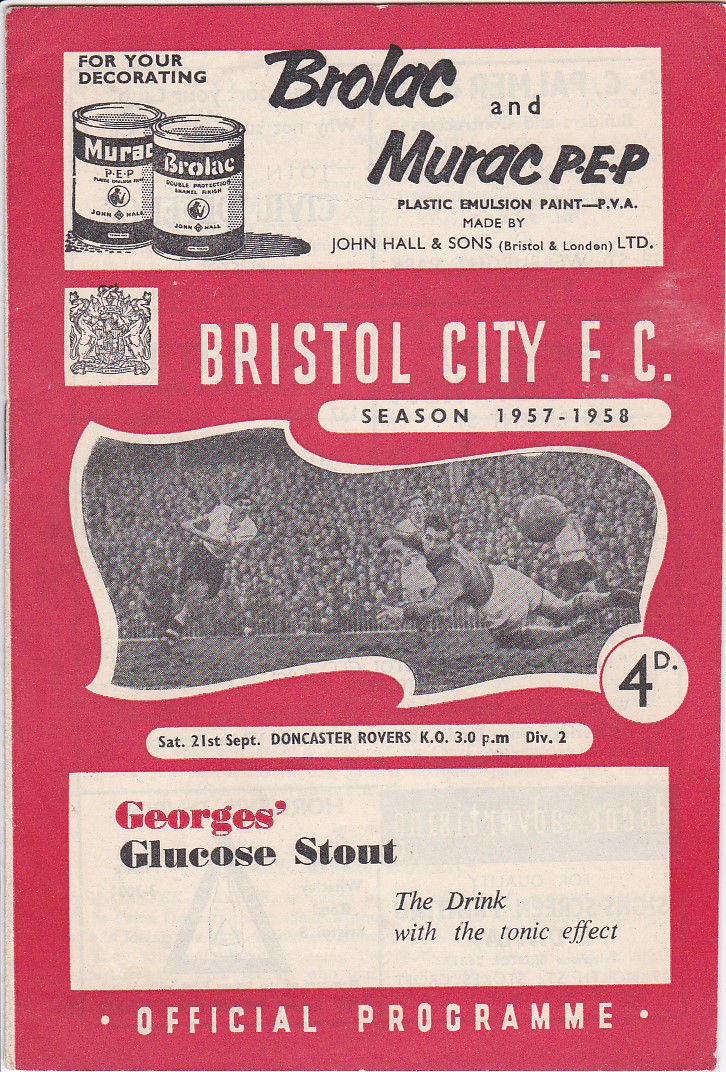The image is an official program poster, presented in portrait orientation with a pink background. It is divided into several distinct sections featuring advertisements and event information. At the top, there is a rectangular advertisement with a white background, showing two paint cans labeled "Brolek" and "Murek PEP Plastic Emulsion Paint PVA," created by John Holland & Sons. Adjacent to the cans, the text reads, "For Your Decorating."

Below this ad, there is event information tied to a football event. The event section features a black and white photograph of a football game from the Bristol City FC 1957-1958 season. The image captures players in action on a football field, with the text "Bristol City FC Season 1957-1958" displayed prominently above it. Additional details include "Set 21st September Doncaster Rovers KO 3pm Dive 2," and another oval-shaped area displaying "4D."

Further down, another white rectangle advertises "George's Glucose Stout, the drink with the tonic effect" in bold letters. Finally, at the very bottom, the text "Official Program" is clearly visible, tying the entire layout together into a cohesive and visually appealing design.